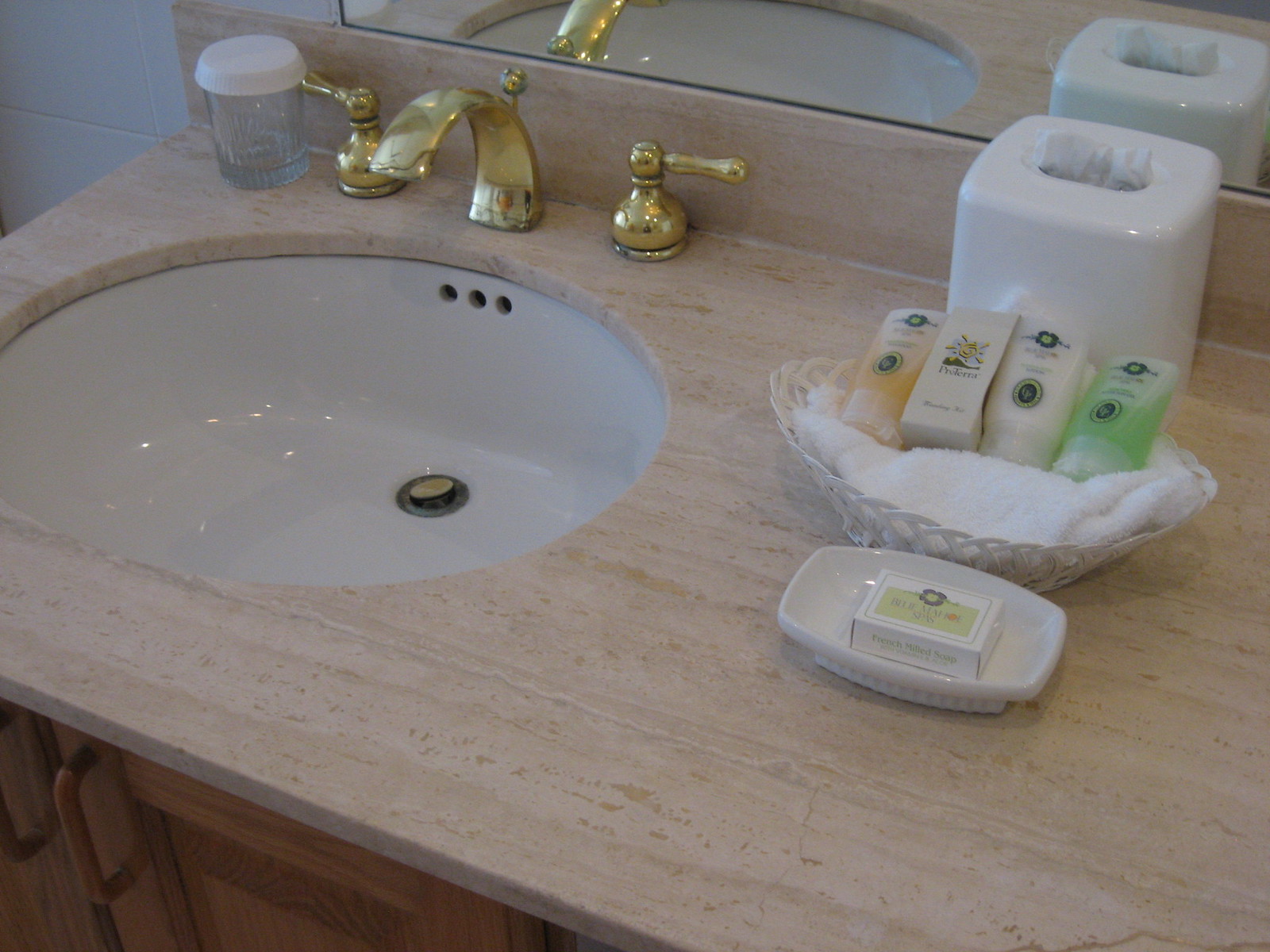This image captures a pristine bathroom sink, prominently featured at the center. The sink is an elegant white porcelain basin seamlessly integrated into a beige marble-like countertop. At the top of the frame, a portion of the wall-mounted mirror is visible, reflecting the understated elegance of the setting. The sink is adorned with gold-colored faucet and handles, adding a touch of luxury.

To the left of the hot water handle, a small glass with a white paper hygiene cover sits neatly, reminiscent of those found in upscale hotel rooms. To the right of the cold water handle, a white tissue holder dispenses tissues while serving as a practical accent. Just in front of the tissue holder is a woven basket filled with amenities typically associated with hotel hospitality: a white hand towel and four travel-sized toiletries. These include a bottle with amber-colored liquid, a small box, and two tubes of liquid — one white and the other green — each likely containing products such as hand wash or face wash.

Below this arrangement, there’s a white porcelain soap dish, holding a miniature-sized bar of soap still encased in its box. The overall setting, with its meticulously arranged amenities and luxurious fittings, exudes both comfort and sophistication, suggesting a high-end or hotel bathroom.